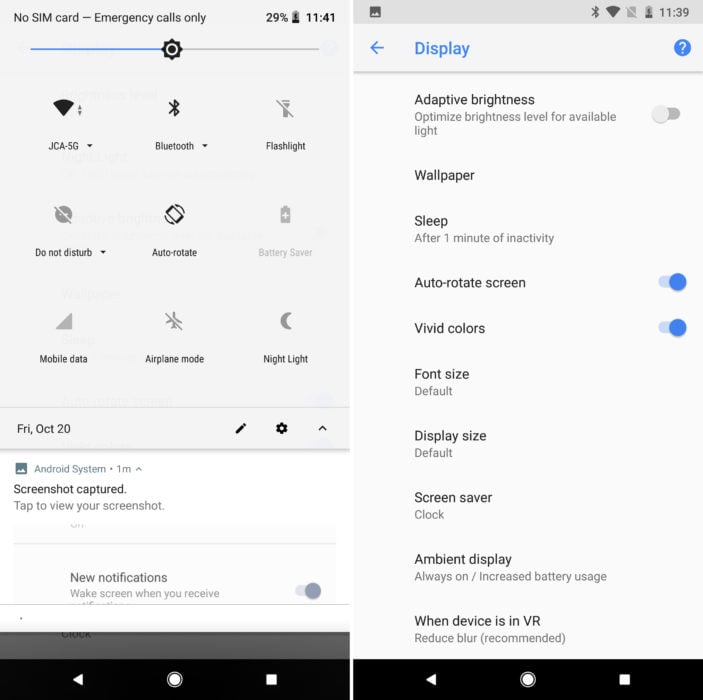The image showcases two Android OS screenshots, each presenting distinct features of the device's interface. 

**Left Screenshot:**
- **Top Bar:** Displays "No SIM card - Emergency calls only," indicating the device lacks a SIM card. The battery percentage is at 29%, and the current time is 11:41 AM.
- **Control Deck:** Includes symbols for brightness control (presumable slider), Wi-Fi, Bluetooth, flashlight, Do Not Disturb, auto-rotate, battery saver, mobile data, airplane mode, and nightlight, all within a drop-down menu accessed via a swipe-down gesture.
- **Notification:** An Android system notification indicates a screenshot was captured one minute ago, with the option to tap and view it.
- **Bottom Section:** Displays the date (Friday, October 20th), an edit icon, a settings cogwheel, and an up-arrow to collapse the menu. A gray notification states that new notifications are turned off.

**Right Screenshot:**
- **Timestamp:** Dated earlier at 11:39 AM, suggesting it was captured before the left screenshot.
- **Top Bar:** Displays Bluetooth and Wi-Fi symbols, along with symbols for a page that is crossed out and a photo.
- **Content Focus:** The primary focus is on various display settings specific to the Android device, emphasizing customization and screen functionality. 

Together, these screenshots depict the user interface and notification management on an Android device, highlighting different aspects of device operation and settings.